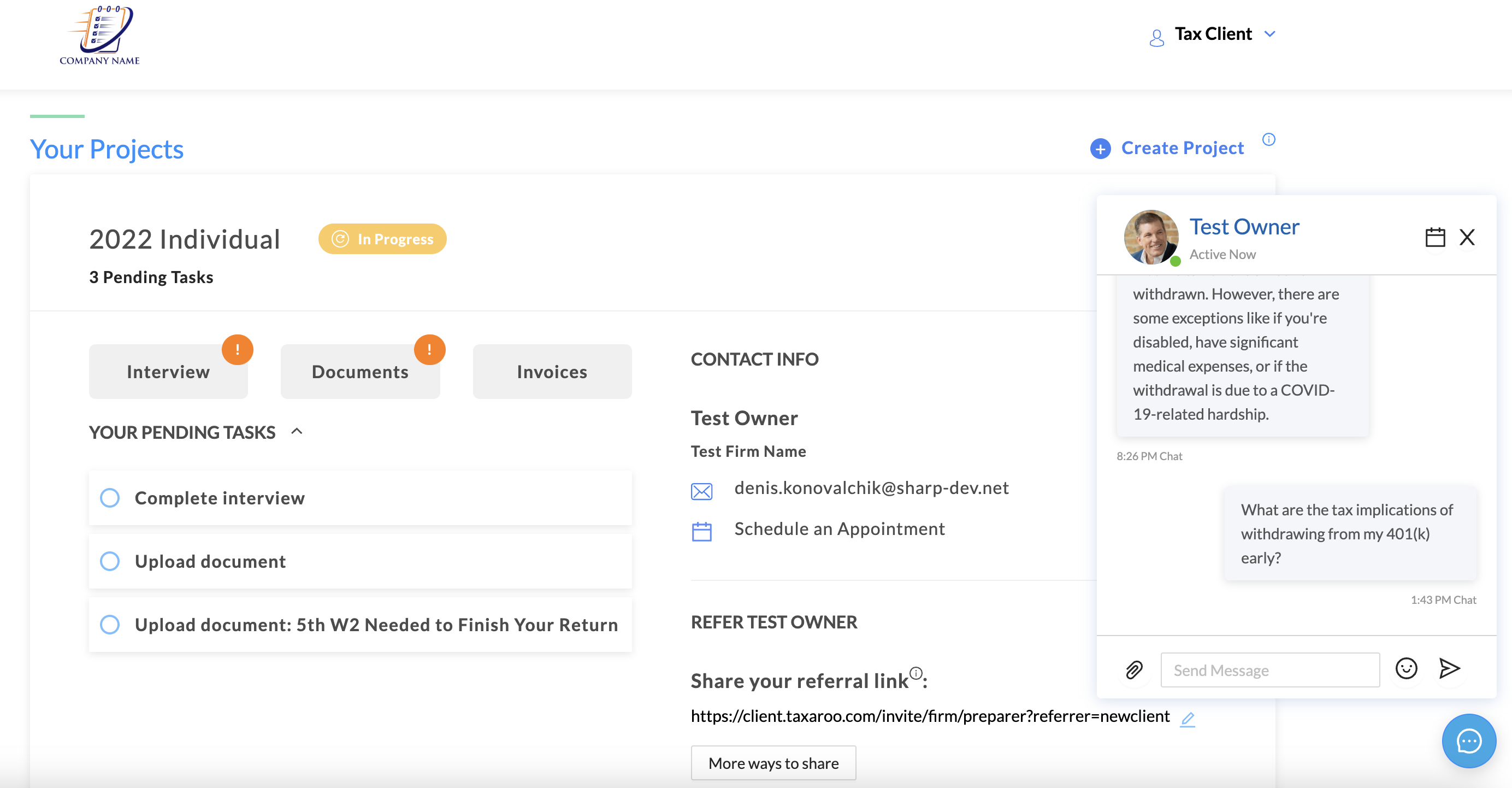A detailed screenshot of a website interface without a visible URL bar is displayed. The top left corner features a cartoon clipboard icon adjacent to the text "Company Name." On the top right, a blue human-shaped icon is paired with the text "Tax Client" in black and a blue drop-down arrow to its right.

A thin gray divider is present below these elements. Directly underneath, on the upper left corner, bold blue letters proclaim "Your Projects." Below this section, in bold black, the text reads "2022 Individual" with a mention of "Three pending tasks." Adjacent to this, an oval orange button with white text states "In Progress."

The next section contains three horizontal gray rectangles with black text. The first reads "Interview," marked with a red dot and a white exclamation mark at the upper right corner. The second rectangle reads "Documents," accompanied by a red-orange dot with a white exclamation mark in the same position. The third rectangle is labeled "Invoices."

Beneath these, the text "Your Pending Task," in bold, is displayed to the left of an upward-pointing arrow. Further below, three blue radio buttons are aligned on the left of respective line sections. Each line item reads, in order: "Complete Interview," "Upload Document," and "Upload Document 5W2 Needed to Finish or Return."

On the right-hand side, a section labeled "Contact Info" includes text: “Test Owner” and “Test Firm Name,” along with fictitious contact information beside blue icons of an email envelope and a calendar. At the bottom of this section, the phrase "Refer Test Owner" appears with a prompt to "Share Your Referral" link below it.

The last column on the far right starts with a blue "Test Owner" label next to a circle icon depicting a middle-aged man. To its right are icons of a calendar in gray and a black X. Text windows, resembling chat exchanges, occupy the space below, featuring white and light gray text bubbles with two exchanged messages. At the bottom of this chat section, there is a rectangular text entry field flanked by a paperclip icon on the left and a gray happy face with a right-pointing arrow on the right.

In the bottom right corner of the interface, a blue circle containing a white speech bubble with three horizontal white dots is visible.